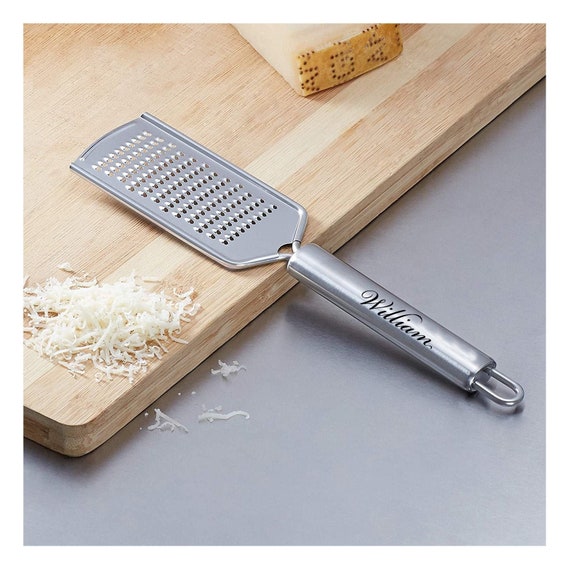The professional product photograph showcases a sleek, functional steel cheese grater designed for commercial use, ideal for an online shop or catalog. The narrow-headed grater features numerous punched holes on its flat, spatula-like surface, effective for finely shredding cheese. Its handle, crafted from polished silver metal, bears the black engraved text "WILLIAM" in a cursive font, evoking a handwritten elegance. The handle culminates in a round silver loop for convenient hanging. The grater is artfully positioned on a wooden cutting board, partially extending onto a grey surface. To its left rests a generous pile of freshly shredded white cheese and to its right, a block of white cheese, suggesting the product's functionality and efficient performance. The well-composed placement and professional quality of the image emphasize the grater's design and practical use.